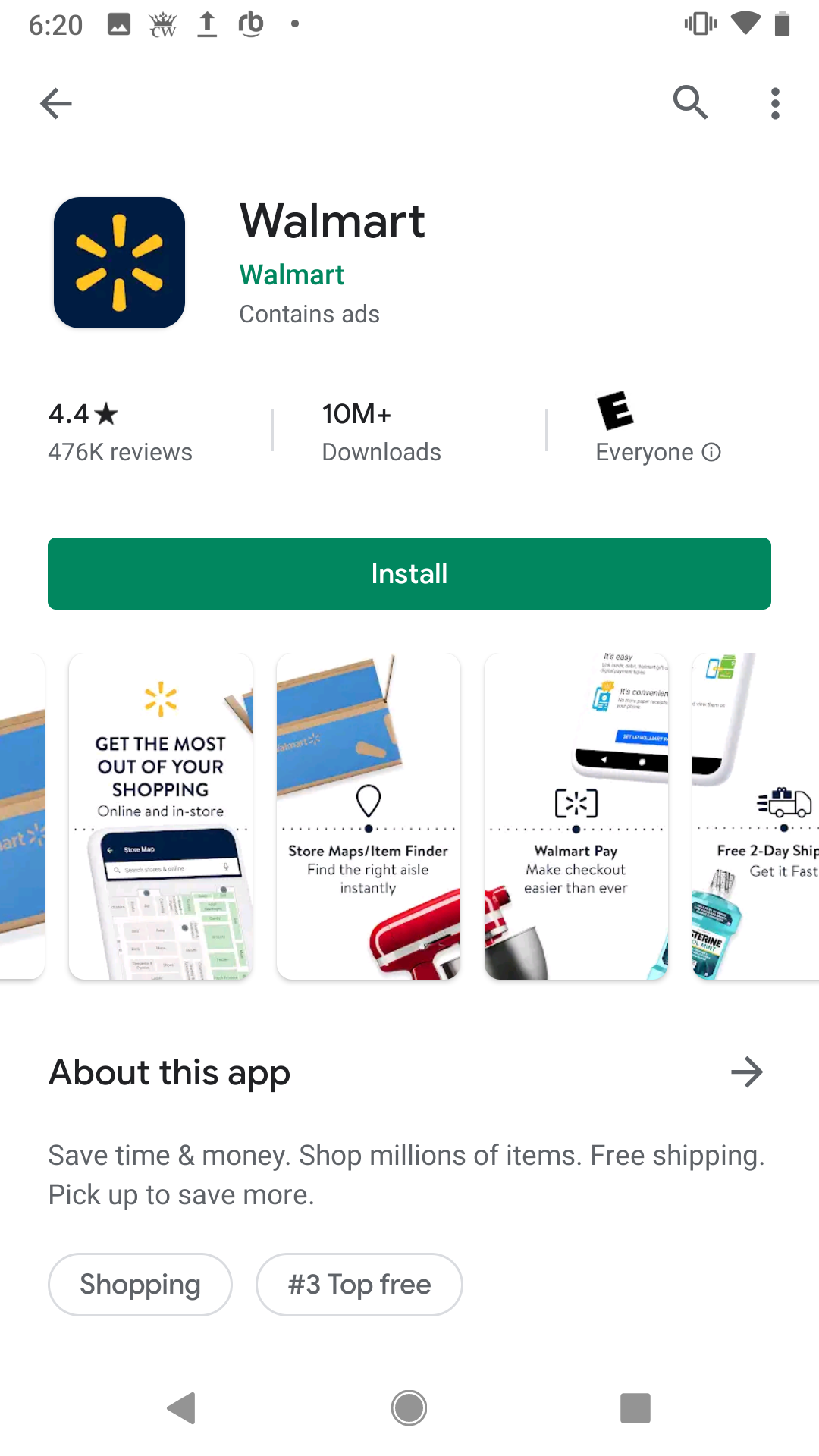This image is a screenshot from a smartphone displaying the Walmart app page. At the top of the screen, indicators show the time, battery percentage, and WiFi status. The app’s title, "Walmart," is prominently displayed, along with a notable 4.4-star rating from 476,000 reviews and over 10,000,000 downloads. It is rated "E for Everyone." 

Below the ratings, a green "Install" button is visible. The screenshot showcases various promotional images of the app. One image highlights, "Get the most out of your shopping, online and in-store," and features functionalities like the store map/item finder, which helps users locate the correct aisle instantly. Another feature, Walmart Pay, is advertised to facilitate easier checkouts. The app also promotes free two-day shipping with images of products such as Listerine and a mixing bowl, alongside Walmart shipping boxes.

At the bottom of the screen, a section labeled "About this app" provides a concise description: "Save time and money. Shop millions of items." Additional benefits are listed, including free shipping and the option to pick up purchases to save more. Tags indicate the app falls under "shopping" and is ranked number three in the "top free" category. The interface includes a back arrow, a gray central circle, and a gray square for navigation. The overall background is predominantly white, contrasted by the dark Walmart logo featuring yellow sun-like lines.